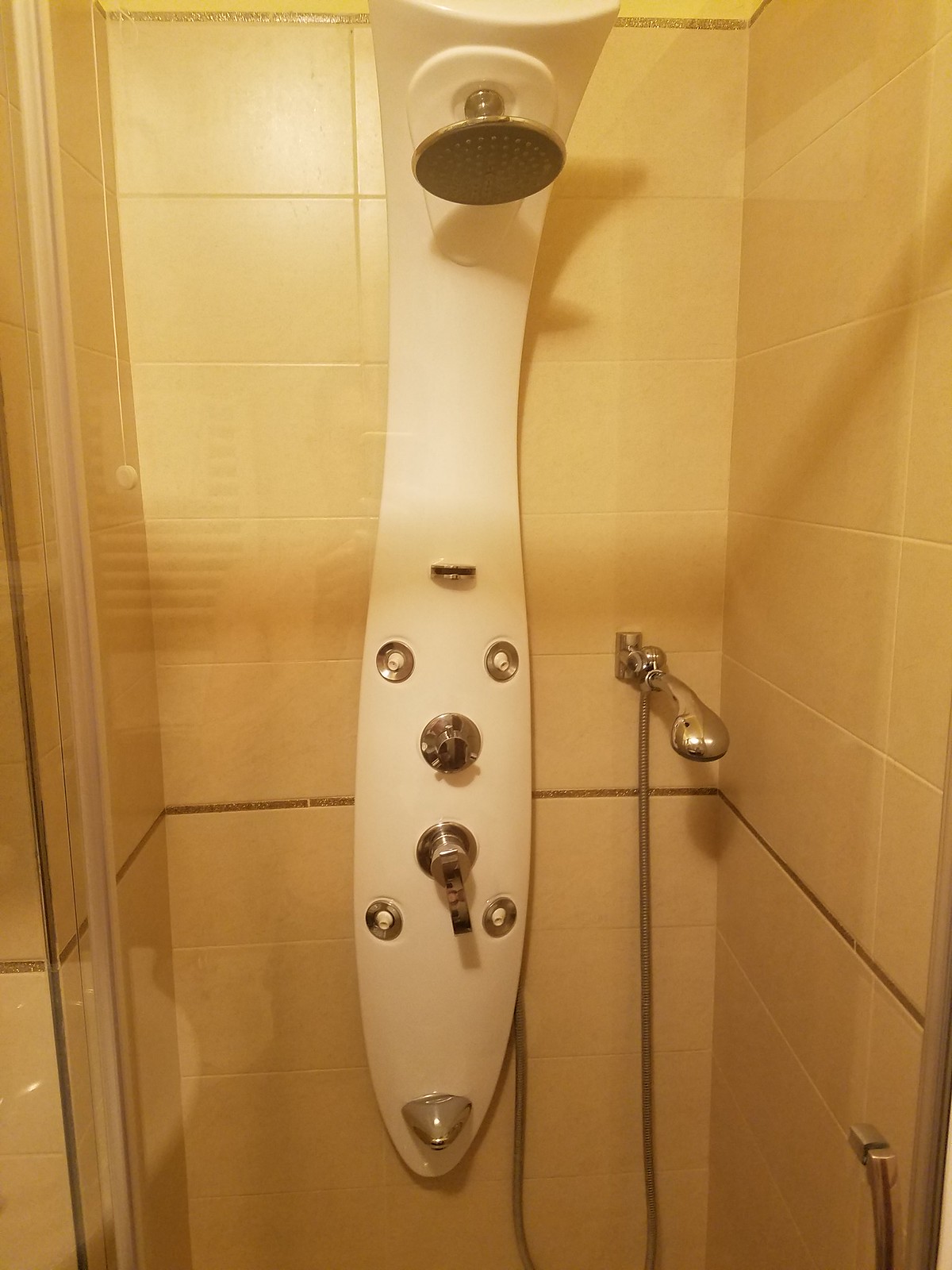This photograph showcases the interior of a small tiled shower cubicle, featuring peach-colored tiles on the walls. Dominating the center of the image is a tall, white stand-up water jet shower system attached to the wall. This system includes several components: a large, flat, circular shower head at the very top for a waterfall-like experience, four jet nozzles evenly spaced along its length, and various silver knobs for adjusting water pressure and temperature.

Adjacent to the main shower system, there is another shower head mounted on a silver metal handle, positioned at about waist level for easy accessibility. This handheld shower head is connected to the wall by a flexible silver hose, allowing it to be used similarly to a hose for targeted water flow. The entire shower cubicle is enclosed by a glass door with a sleek, silver-colored handle, completing the modern and functional design.